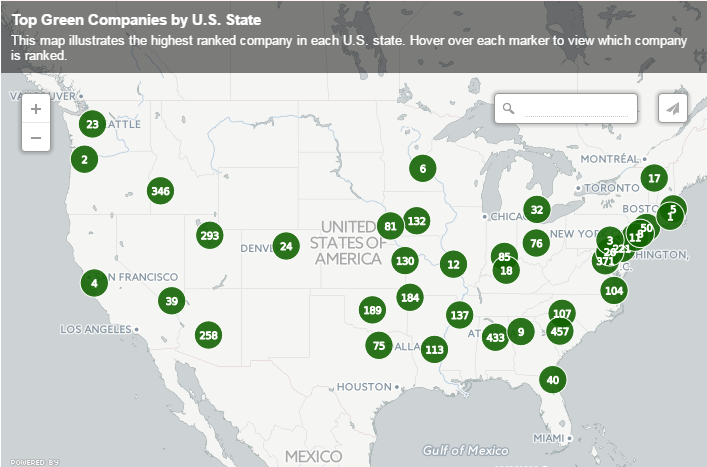This PC screenshot showcases a simplified map of the United States, highlighting the top green companies by state. White text across a gray border at the top of the map reads, "Top Green Companies by U.S. State." Below this title, additional text explains that hovering over each green circle marker reveals the highest-ranked green company in that state.

The map is minimalist with faint blue outlines delineating state borders, and the oceans rendered in a very pale blue hue. Green circles of varying sizes, each marked with a white number, are distributed across the map. The eastern United States is densely populated with these markers, particularly along the East Coast, indicating a higher concentration of top green companies in this region. In contrast, fewer markers appear across the western U.S. and along the West Coast.

Massachusetts is marked as number one, signifying it has the highest-ranked green company, while California holds the fourth spot. Users can interact with the map by clicking on the numbered markers to uncover more information about each state's leading green company.